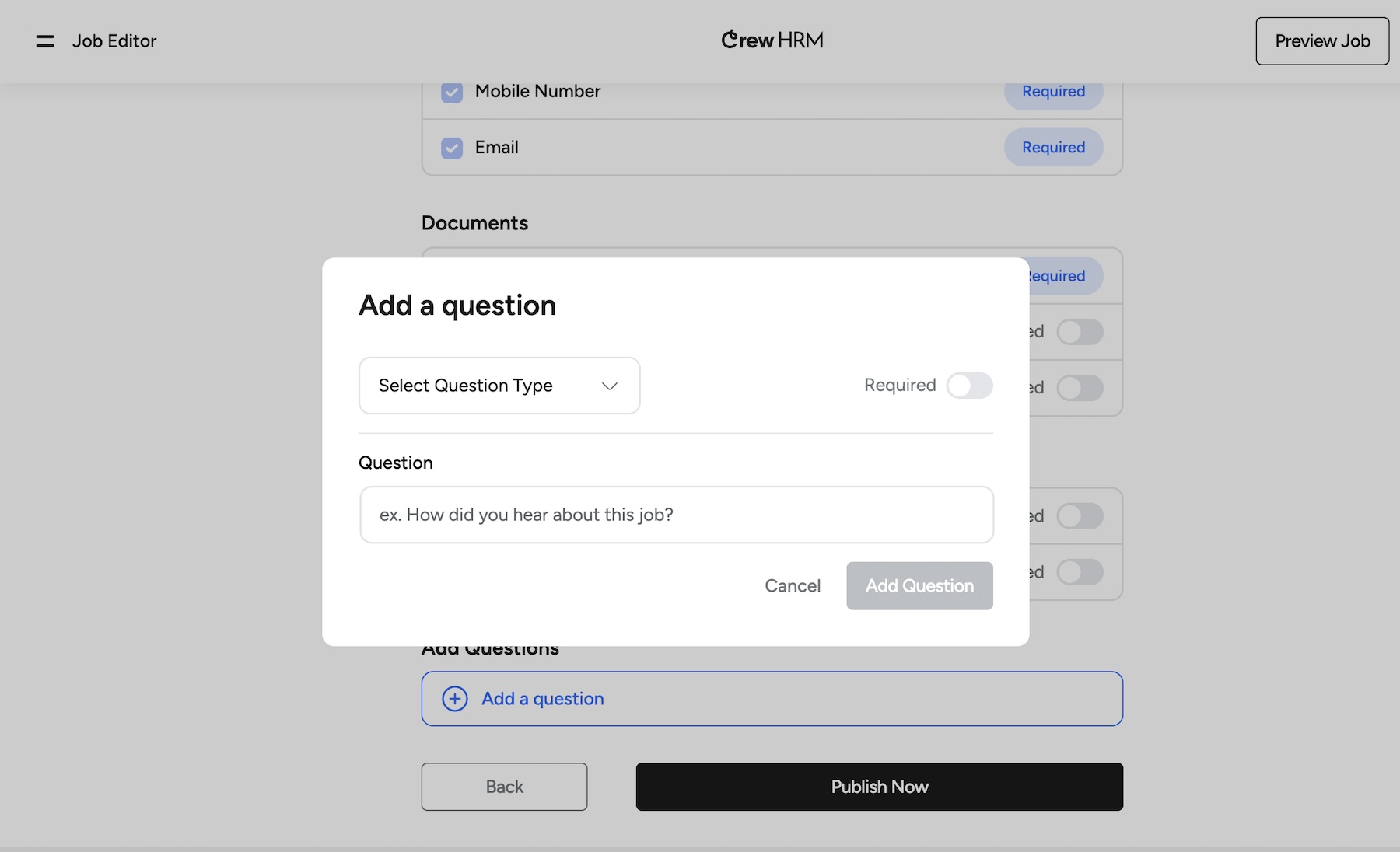The screenshot features an HR software interface, specifically within a "Job Editor" page. The main webpage is partially obscured by a central pop-up box, leaving some interface elements visible. 

At the top left of the visible webpage, "Job Editor" is prominently displayed in black font. Centrally, the title "Crew HRM" is visible, and on the right, it initially reads "Preview Job" (corrected from "previous job"). Below this section, visible fields include "Mobile Number" and "Email," though further details are concealed by the pop-up box.

The pop-up box, a white rectangle, starts in the upper left corner with the text "Add a Question" in black font. Below this text is a dropdown menu labeled "Select Question Type," followed by a field labeled "Question," with an example prompt: "Ex: How did you hear about this job?" Two buttons, "Add Question" and "Cancel," are present, though they require input to be activated.

Returning to the main webpage layout, there is another option to "Add a Question." At the bottom of the visible section of the webpage, a black rectangle contains the text "Publish Now" in white font, indicating a final action button for publishing changes.